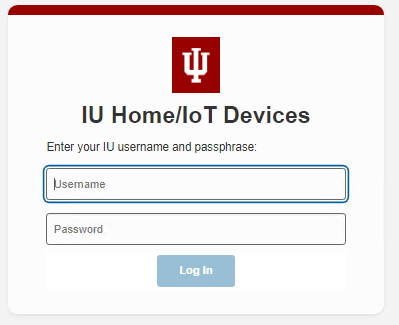The image depicts a user interface for an IU Home/LOT application. The background is shaded gray, and a white square is superimposed over it, creating a shaded gray border around the white area. At the top of the white square, there is a dark red border. Below this border, a dark red square contains an icon, displaying a white trident emblem as the logo.

Further down, there is a section of white space followed by bold black text: "IU Home/LOT Devices," with "IU," "H," "T," and "D" capitalized. Beneath this text, in smaller print, it instructs users to "enter your IU username and passphrase."

Below the instruction, there is a blue-outlined box labeled "Username" and a black-outlined box labeled "Password." Finally, at the bottom, there is a light blue rectangle with the text "Log In."